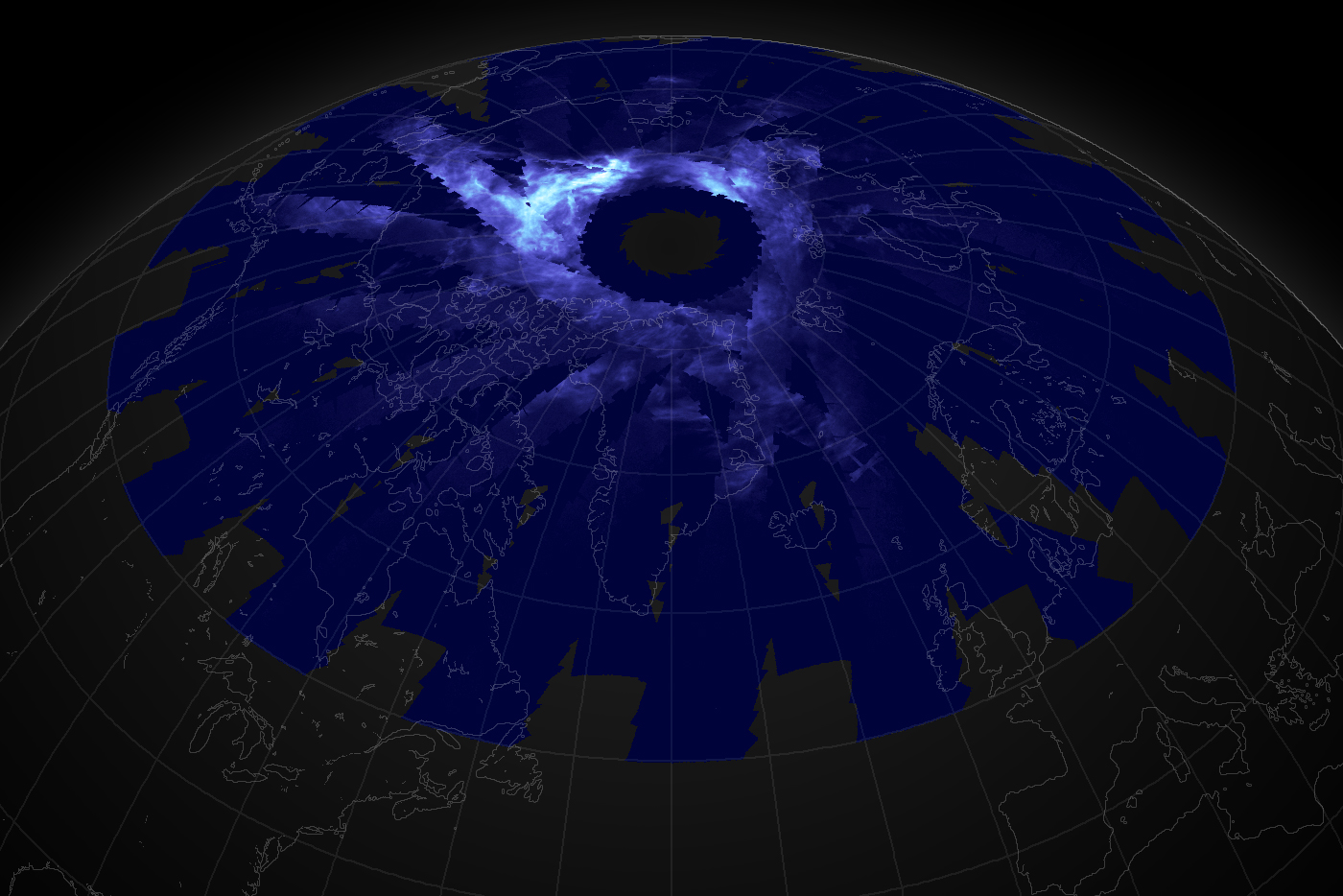This image is a graphic representation of Earth viewed from above, focusing on the North Pole with a black background. The upper portion of the image features a prominent black circular blurb, possibly representing a black hole or a dark cloud, surrounded by a dark navy blue sky with wispy, white cloud-like formations. The Earth is depicted with discernible continent outlines, including the United States to the bottom left and Europe to the bottom right. The globe contains visible longitude and latitude lines, and the landmasses are depicted in varying hues of green, suggesting vegetation. The dark setting, combined with Earth's white circumscribed outline, contrasts sharply against the black backdrop. The visual intricacy includes what appears to be overlays or cutouts that resemble building silhouettes. This highly detailed image merges both elements of realism and artistic interpretation, detailing the Earth's curvature, landmasses, and atmospheric phenomena.